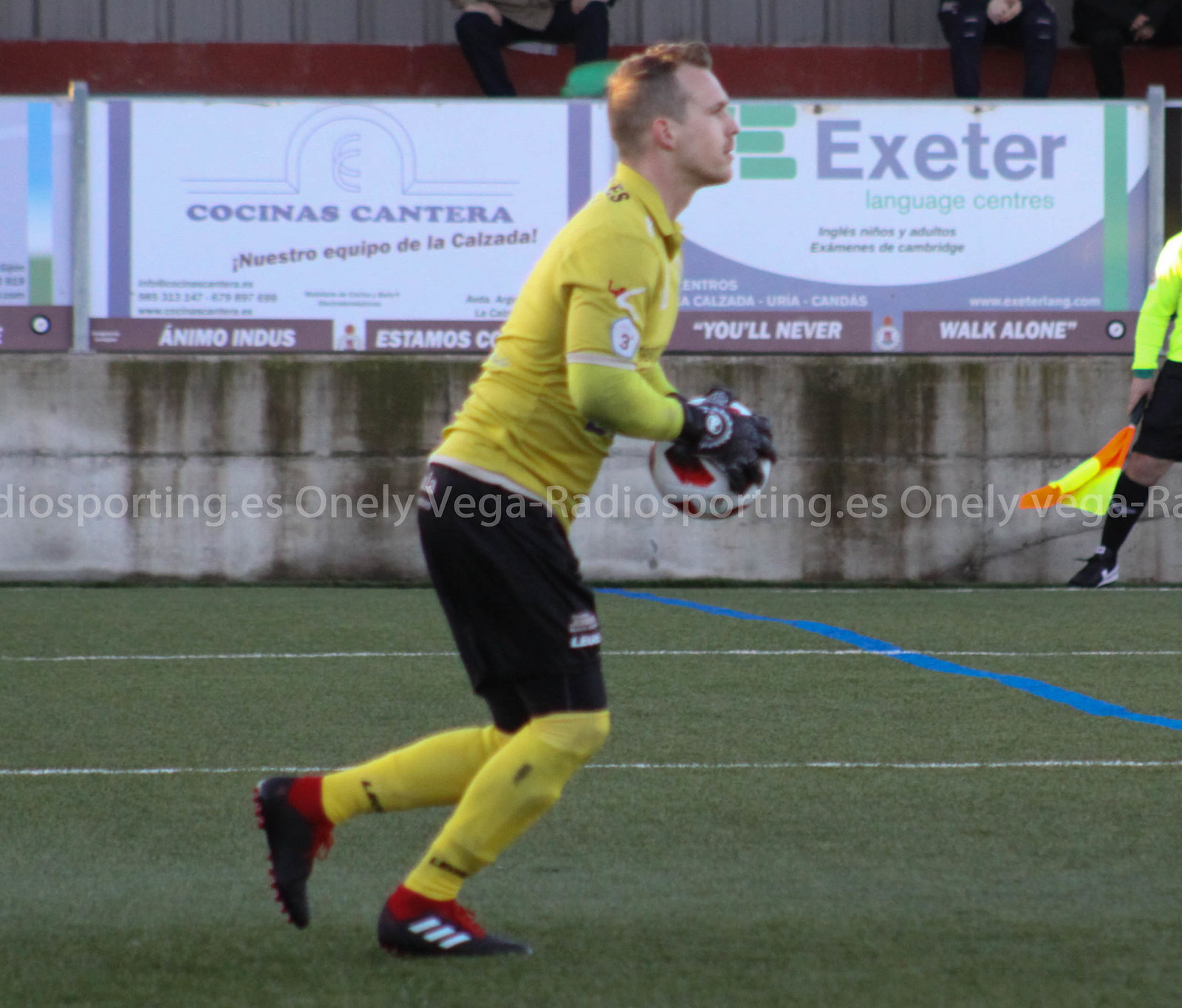In this image, a soccer player, likely in his late 20s to early 30s, stands ready to throw a soccer ball. He is dressed in a yellow uniform consisting of a long-sleeve jersey and matching leggings. He also sports black shorts, black and white cleats with red laces, and red socks. A brace is visible underneath his attire, indicating preparation for rigorous activity. The player has short cropped hair and a slight stubble, emphasizing his athletic build.

He holds a soccer ball marked with red and black graphics against a white backdrop. The scene is set on green AstroTurf within an indoor practice venue. Behind the player, several elements are visible including a concrete wall adorned with sponsor banners for Exeter Language Centers and Cocinos Cantera. The wall shows visible water stains, and a few spectators can be seen seated in the background.

Also in the frame is a partially obscured referee on the right side, wearing a bright green long-sleeve jersey, black shorts, and black leggings, holding an orange and yellow flag. A watermark across the image reads onlyvegaradiosporting.es, hinting at the source of the photograph.